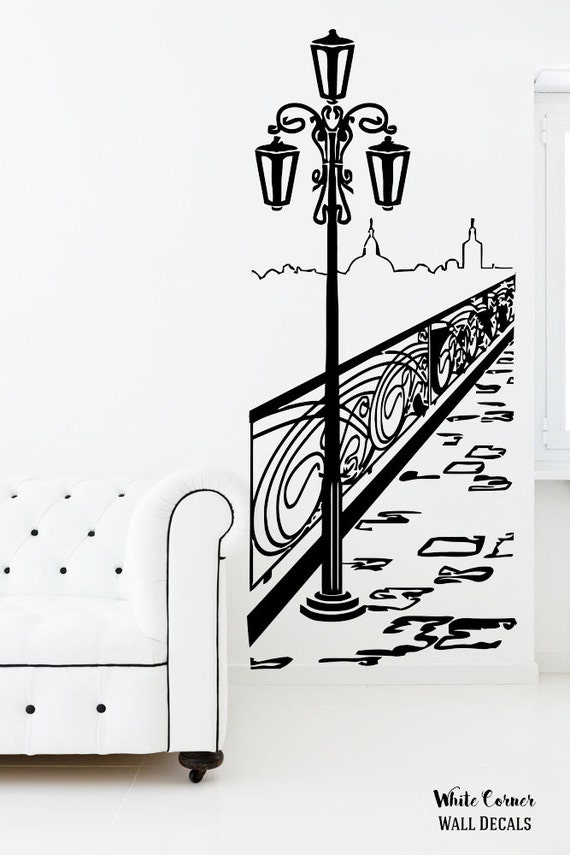This vertical rectangular advertisement showcases a striking monochrome wall decal in a minimalist setting. The background features a very light gray or white wall and floor. In the bottom left corner, there is the partial visible side of a sleek white sofa with black buttons and trim, extending off the left side of the image. Notably, the armrest and a small cylindrical protrusion or leg are visible underneath the sofa. 

To the right of the sofa, the wall decal dramatically depicts an urban street scene in black and white. This detailed illustration includes a railing with intricate metal designs extending up and to the right, a street lamp with three lights (two lateral and one on top), and what appears to be a cobblestone walkway or bridge. The cityscape and architectural elements in the decal give an illusion of depth and add an artistic touch to the setting. The bottom right corner of the image prominently displays the text "White Corner Wall Decals," underscoring the product being advertised.